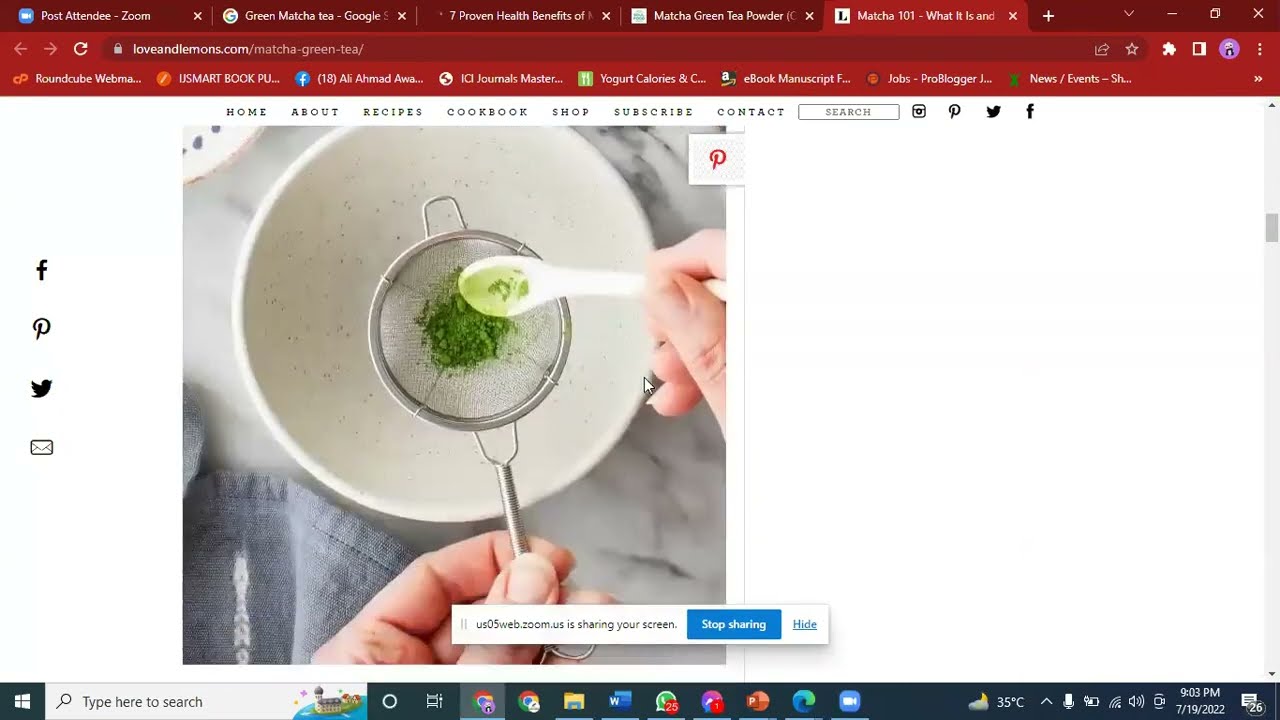The image displays a detailed screenshot of a computer screen featuring an open internet browser with multiple tabs. Prominently, the first tab reads "Post Attendee Zoom," followed by "Green Matcha Tea Google," "Seven Proven Health Benefits Of," "Matcha Green Tea Powder," and "Matcha 101 What It Is And." The browser is displaying a web page with a mainly white background, likely part of a cooking website, as suggested by text references to "stop sharing recipes," "home," "about," and "cookbook," implying a focus on culinary content.

Central to the webpage is a photograph depicting a detailed scene involving matcha tea. The image features a white teacup on a cloth-covered table. Above the cup, two hands are positioned. The left hand is holding a silver ladle containing green matcha powder, while the right hand holds a small spoon with remnants of the powder. The setting appears methodical, indicative of matcha preparation with an attention to detail highlighting the culinary process. The overall theme is enhanced by the contrast of the green matcha against the white cup and background, suggesting a meticulously curated cooking website.

Additionally, the computer screen's typical Windows interface elements are visible, including a horizontal strip at the bottom with a dark green hue characteristic of either Windows 10 or 11, containing various application icons, a search bar to the left, and system information to the right.